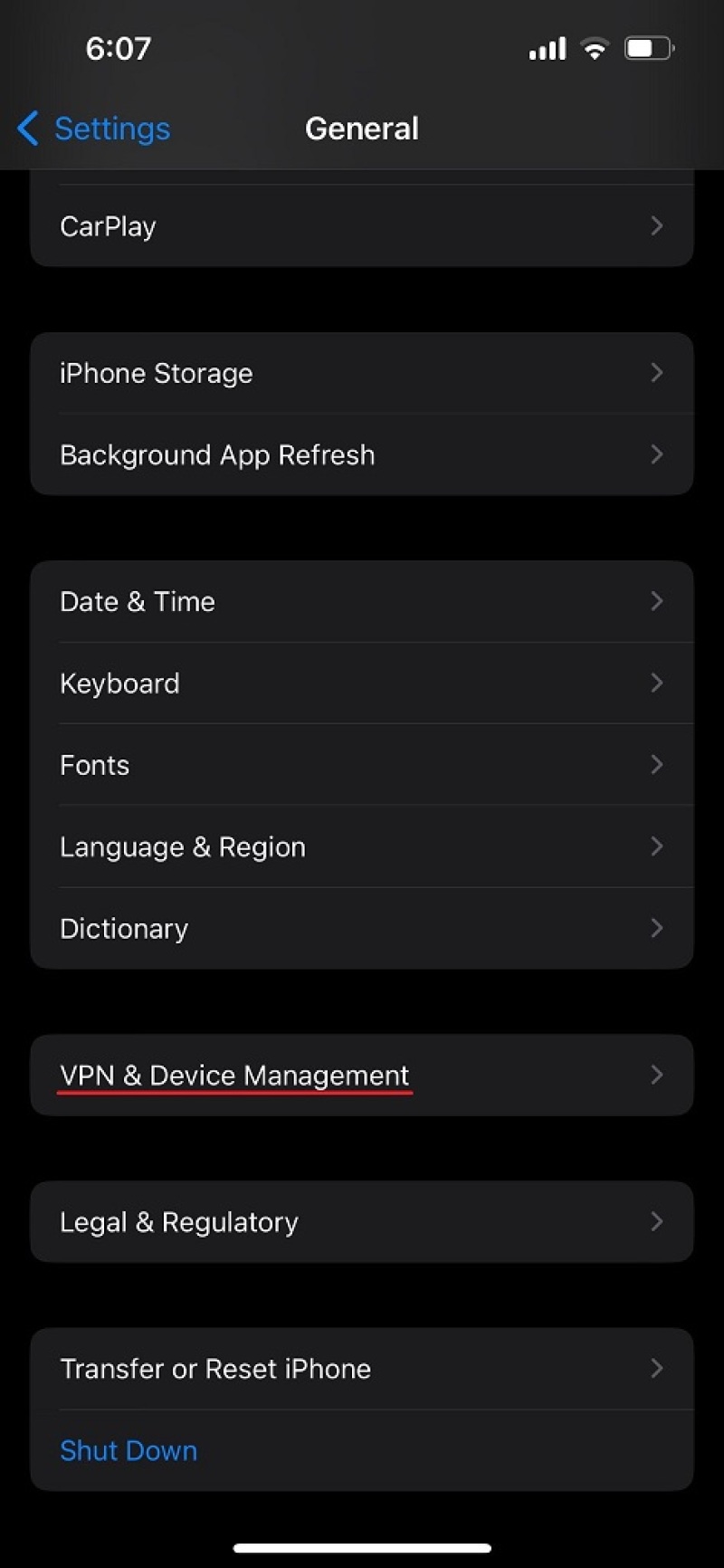**Screenshot Description**:

This image is a screenshot of a settings page on a smartphone.

- **Header**: 
  - The top section features a dark grey header. 
  - On the top left, white numerals read “607.”
  - On the top right, there are three status icons.
- **Navigation Elements**:
  - In the bottom left of the header, blue text indicates "Settings."
  - Beside this text, there is a blue arrow pointing to the left.
  - In the bottom center of the header, white text reads “General.”
- **Body**:
  - The main body of the page has a black background.
  - The content is arranged in panels of dark grey rectangles with rounded corners.
- **Panels**:
  - **Top Panel (Partially Visible)**:
    - Near the top, a thin light grey line runs almost the entire width.
    - Bottom left corner: white text reads "CarPlay."
    - Bottom right corner: a light grey arrow points to the right.
  - **Second Panel**:
    - Composed of two rows:
      - First row: "iPhone Storage."
      - Second row: "Background App Refresh."
  - **Third Panel**:
    - Contains five rows:
      - "Date & Time."
      - "Keyboard."
      - "Fonts."
      - "Language & Region."
      - "Dictionary."
  - **Fourth Panel**:
    - Single row with underlined text: "VPN & Device Management."
  - **Fifth Panel**:
    - Single row: "Legal & Regulatory."
  - **Sixth Panel**:
    - Two rows:
      - "Transfer or Reset iPhone."
      - The final row features blue text: "Shut Down."

Each panel is separated by thin grey lines and small sections of the black background, maintaining a neatly structured appearance.